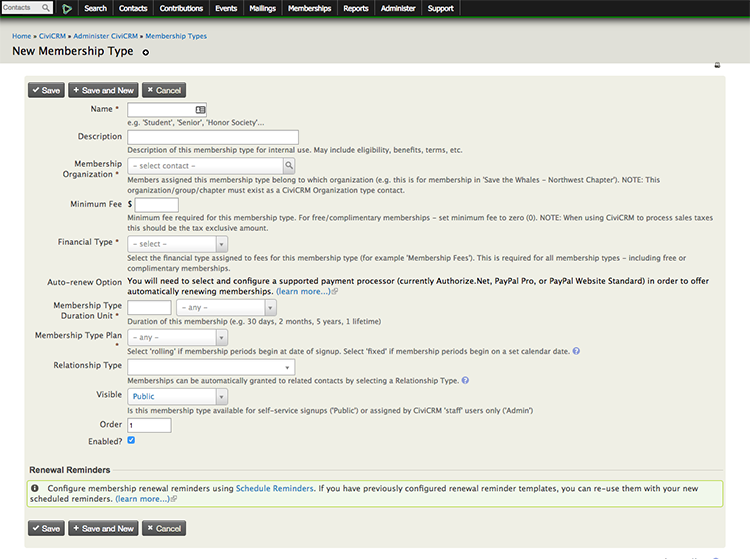The image showcases a section of a website devoted to adding a new membership type. While the name of the website is not visible, the menu bar at the top of the image is prominently displayed. This menu bar, stretching horizontally from left to right, is black and hosts various navigational options.

On the left side of the menu bar, there's a search bar labeled "Contacts." Adjacent to this, a green symbol resembling a play button is present. Following the symbol, the menu features several clickable options in sequence: "Search," "Contacts," "Contributions," "Events," "Mailing," "Membership," "Reports," "Administrator," and "Support."

Below this menu, the primary focus of the image is a tree-like structure that lists various membership types. The text "New Membership Type" is clearly visible. Below this heading, there is a form with multiple fields available to fill out. The form fields include:

- Name
- Description
- Membership Organization
- Minimum Fee
- Financial Type
- Auto-Renew Options
- Membership Type Duration Unit
- Relationship Type Option

This descriptive setup allows users to configure specifics for a new membership type within the website's interface.